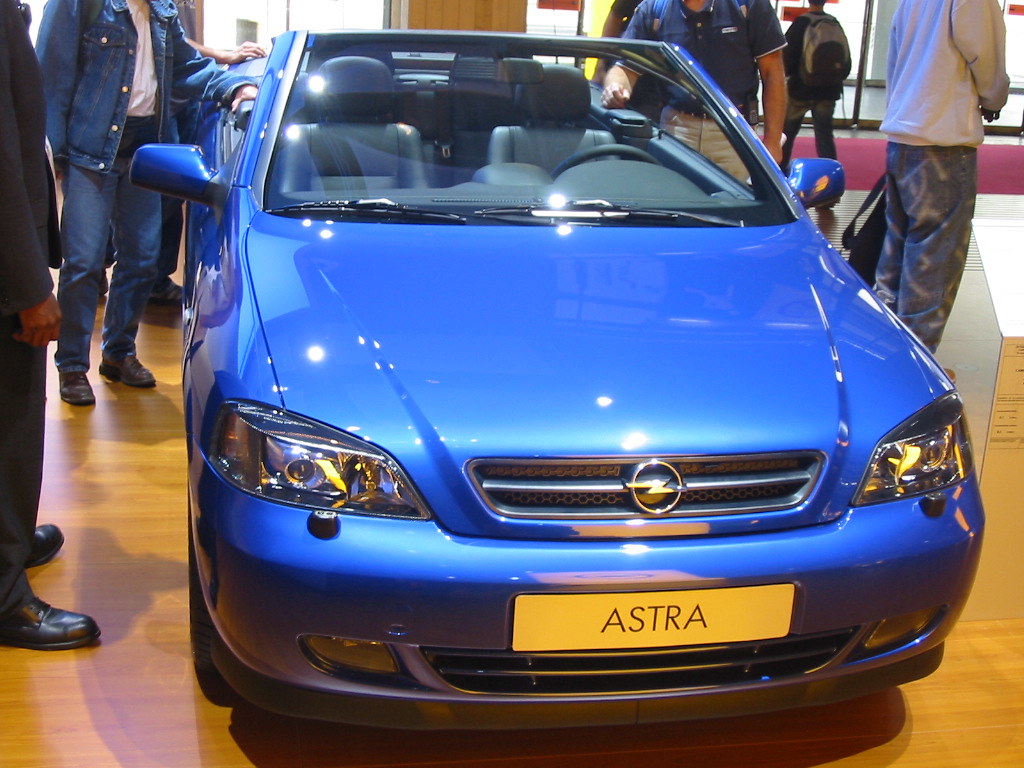The image depicts a deep blue convertible car, brand new and seemingly on display at a car show or dealership. The car has a sleek design with clear headlights, a small grille featuring a lightning bolt logo, and an orangish-yellow tag in the front that reads "Astra" in thin black letters. It boasts a luxurious black leather interior, clearly visible with the top down. The car is parked on a hardwood floor inside a room, illuminated by overhead lighting. Surrounding the car are multiple people, primarily men, casually dressed with some wearing jeans and jackets, one possibly in business attire indicative of an auto dealer. The individuals are engaged with the car, some with hands on it, indicating their interest in this impressive vehicle.